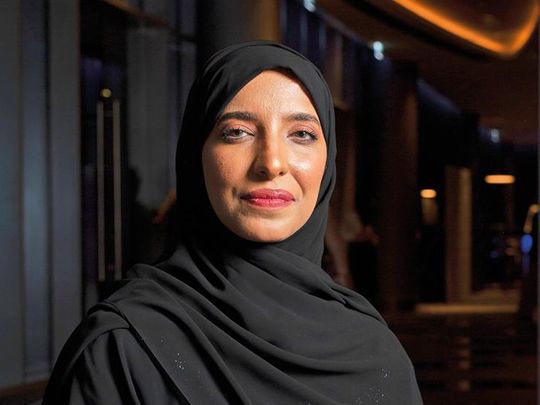In the image, we see a Muslim woman dressed in a black hijab that is wrapped tightly around her head and draped across her chest from right to left. She is posed directly facing the camera with a slight, pressed smile, showing no teeth. Her makeup is noticeable, featuring pink lipstick, full-on foundation, blush, well-defined eyebrows, mascara, and eyeshadow, giving her a polished appearance. The background is slightly blurred but appears to place her indoors, with faintly visible columns behind her and lighting that illuminates her left side. The overall color scheme includes black, pink, and various shades of brown, yellow, and white. There is no text on the image and it could be a profile or headshot photo, showcasing her serene yet captivating expression.